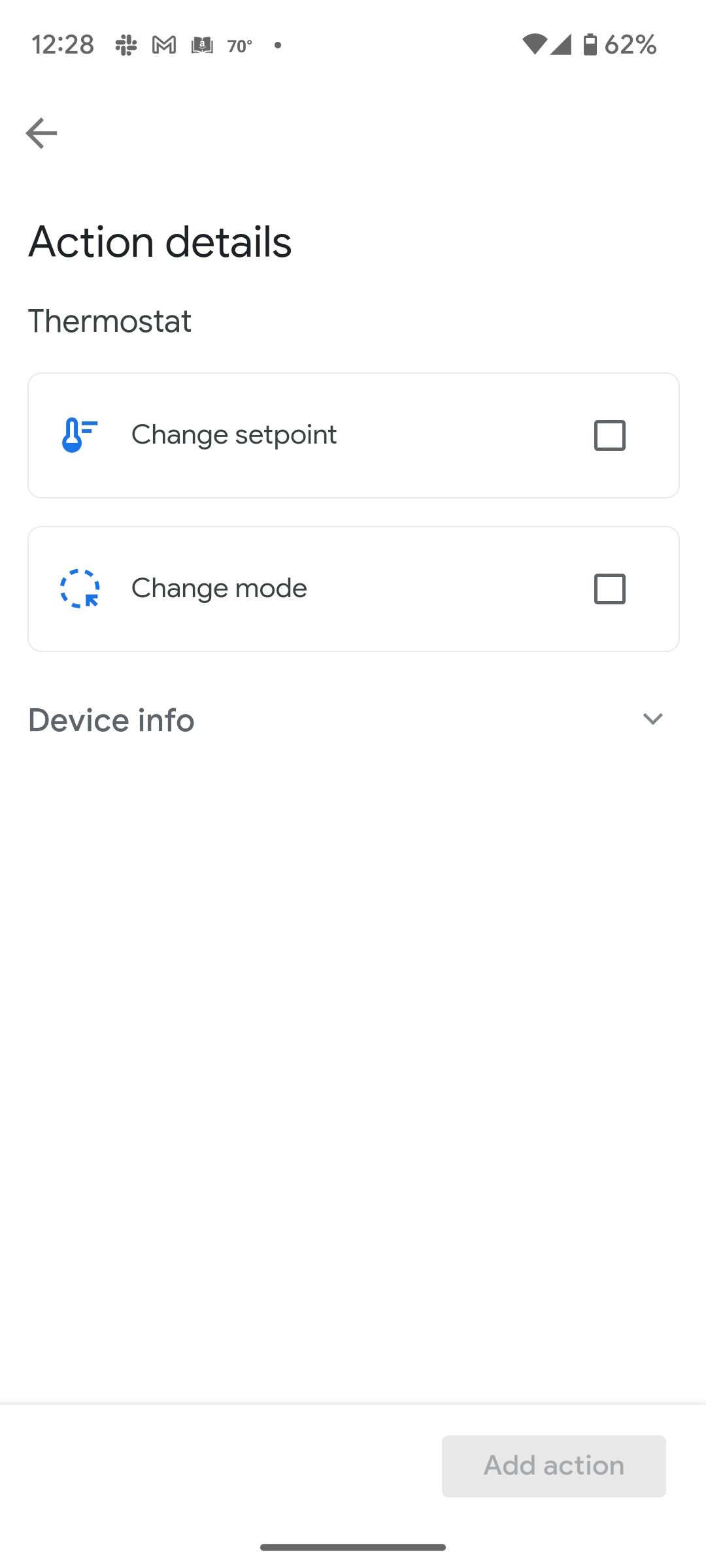The screenshot depicts a user interface with a predominantly white background. At the very top, the time is displayed as 12:28, accompanied by a series of notification icons: a cross symbol, a Gmail icon, a book-like icon, and the temperature reading of 70 degrees Fahrenheit. To the far right, icons indicate the Wi-Fi signal strength and a 62% battery level.

Below this status bar, on the left side, is a left arrow key, followed by the action details. Beneath this, the title "Thermostat" is displayed. Lower down are two light gray-bordered boxes:

1. The first box features a blue thermostat icon with the label "Change Set Point" next to it, and includes a checkbox for selection on its right.
2. The second box contains a dotted circle icon with the label "Change Mode" beside it, which also has a corresponding checkbox to the right.

Under these boxes, on the left side, the text "Device Info" appears, and to its right is a downward arrow button, indicating a drop-down menu.

The lower part of the image remains solid white, with a light gray horizontal line near the bottom. Beneath this line, to the right, is a box labeled "Add Action."